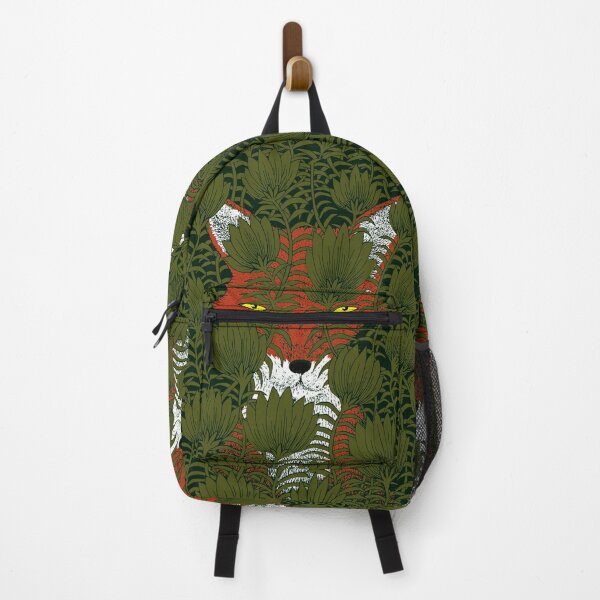The image depicts a green and black backpack with long dangling straps, hanging from a small, curved wooden hook attached to a white wall. The backpack, which is rounded at the top and squared at the bottom, features a detailed pattern of green leaves and flowers. Concealed within this foliage is an artfully camouflaged fox—orange and white with yellow eyes, orange-tipped ears, and a white chest and mouth. The fox appears to be peeking out from the foliage, blending seamlessly with the green background, creating an intricate and captivating design on the backpack.